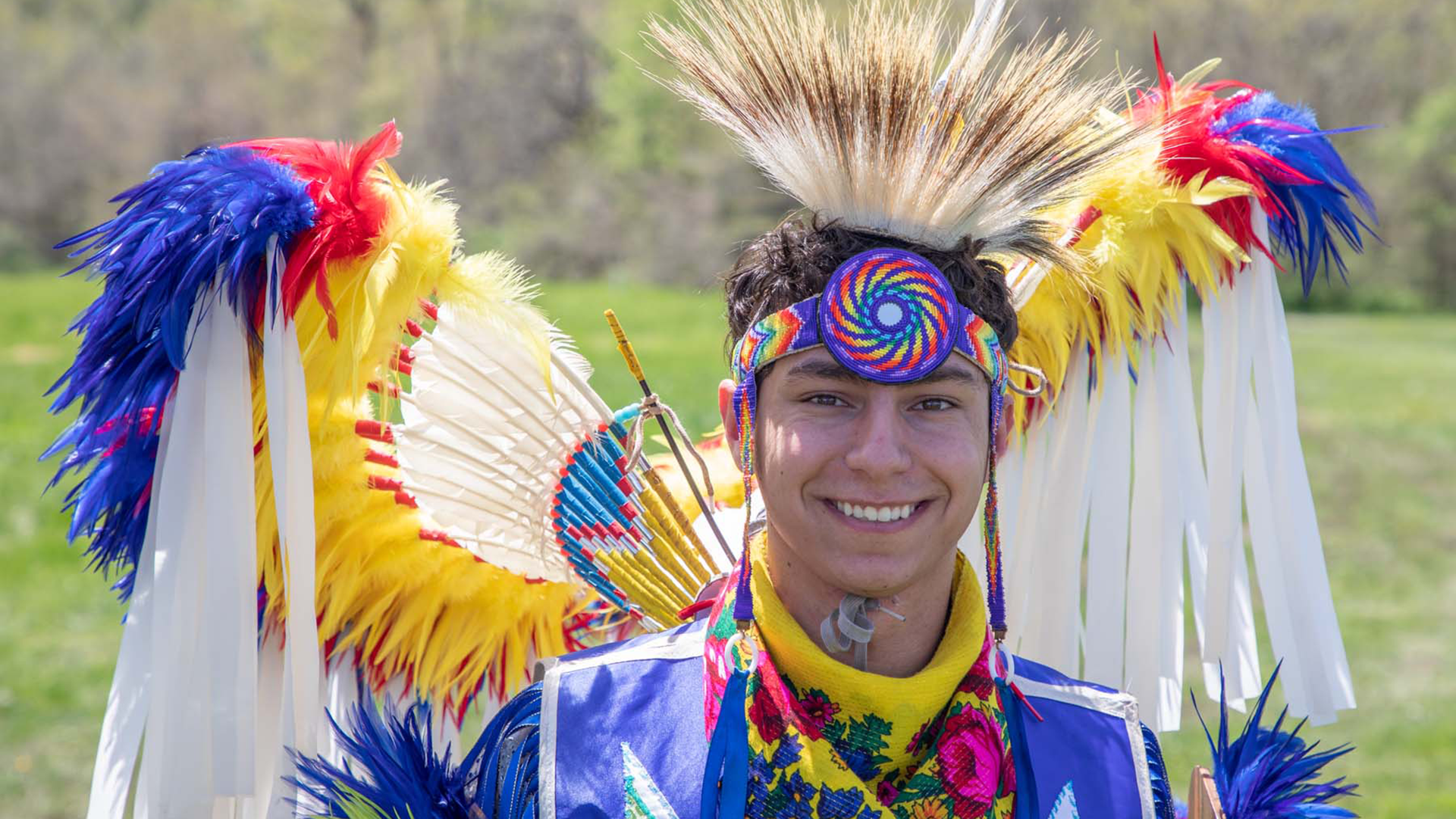In the photograph, a young man, likely in his early 20s, is smiling warmly at the camera. He sports a tan complexion and short, messy black hair adorned with a headdress reminiscent of traditional Native American attire. The headdress appears to be crafted from animal fur, dark brown at the top and transitioning to white at the bottom, with a rainbow-colored beaded headband featuring a spiral design at its center.

He is dressed in a vibrant and colorful outfit, dominated by shades of blue but also incorporating significant amounts of yellow, red, and white. A yellow scarf with an intricately embroidered floral design drapes around his neck. His sleeves are blue with sharp blue shards resembling pieces of paper, and striking feathers embellish the sides. 

Prominent large wings extend from his back, constructed from long white strips of cloth with blue, red, and yellow feathers at the ends, giving the ensemble a dramatic and ceremonial flair. The background shows a lush green field with trees, indicating a natural outdoor setting. The overall attire suggests a richly detailed and ritualistic Native American costume, filled with cultural symbolism and colorful artistry.